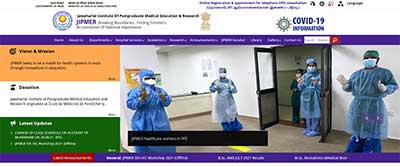**Detailed Caption:**

The image depicts the cover of a report or brochure related to COVID-19, primarily written in Chinese. The layout includes various colored boxes with text. An orange box contains information on "views and missions," while a green box below apparently has some enigmatic content. Unfortunately, due to the text being in Chinese and the image's blurriness, the details are difficult to decipher. The central part of the cover showcases a photograph of an empty ER (Emergency Room). Medical personnel are seen standing, donned in full protective gear including masks, hair covers, and hazmat suits, embodying precautionary measures against the virus. The report's name, "Jip-meh," is also visible along with an emblem and an image of a gear, reinforcing the document's thematic focus on "COVID-19 in population."